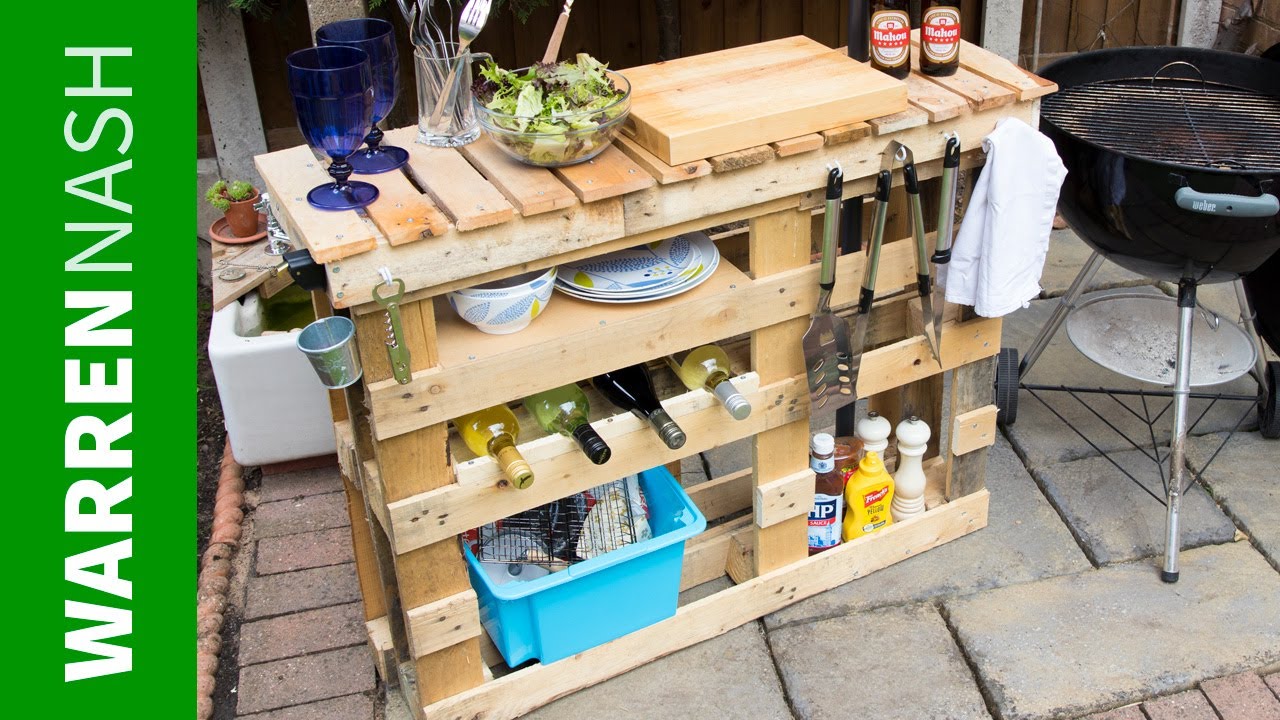In this detailed image, we see a homemade outdoor bar and prep station set against a patio with concrete flooring and surrounded by brickwork. On the left side of the image, there's a green banner with bold white block letters spelling "Warren Nash." The bar itself appears to be fashioned from unfinished pallet wood, with visible raw slats and no varnish or paint. 

On the top surface of the bar, there is a wooden cutting board, a clear glass salad bowl filled with a green salad, a clear glass mug containing various utensils including forks and spoons, and two transparent cobalt blue goblet glasses. Toward the far right of the top counter stand three beer bottles.

The bar features multiple shelves: the second shelf holds stacked plates and bowls, the third contains four wine bottles laid on their sides, and the bottom shelf houses a sky blue plastic tote box filled with miscellaneous items. Further, there is a range of condiments, including a yellow mustard container, a bottle of barbecue sauce, and salt and pepper shakers.

Attached to the side of the bar nearest the grill are hooks holding barbecue utensils like tongs, a spatula, and a white towel. To the right of the bar is a black Weber kettle grill, with its lid set off to the side, showing the grate and three metal legs. In the background, there is a hint of a cooler or planter, additional wooden elements, and what looks like the exterior of a house, completing the backyard barbecue setup.